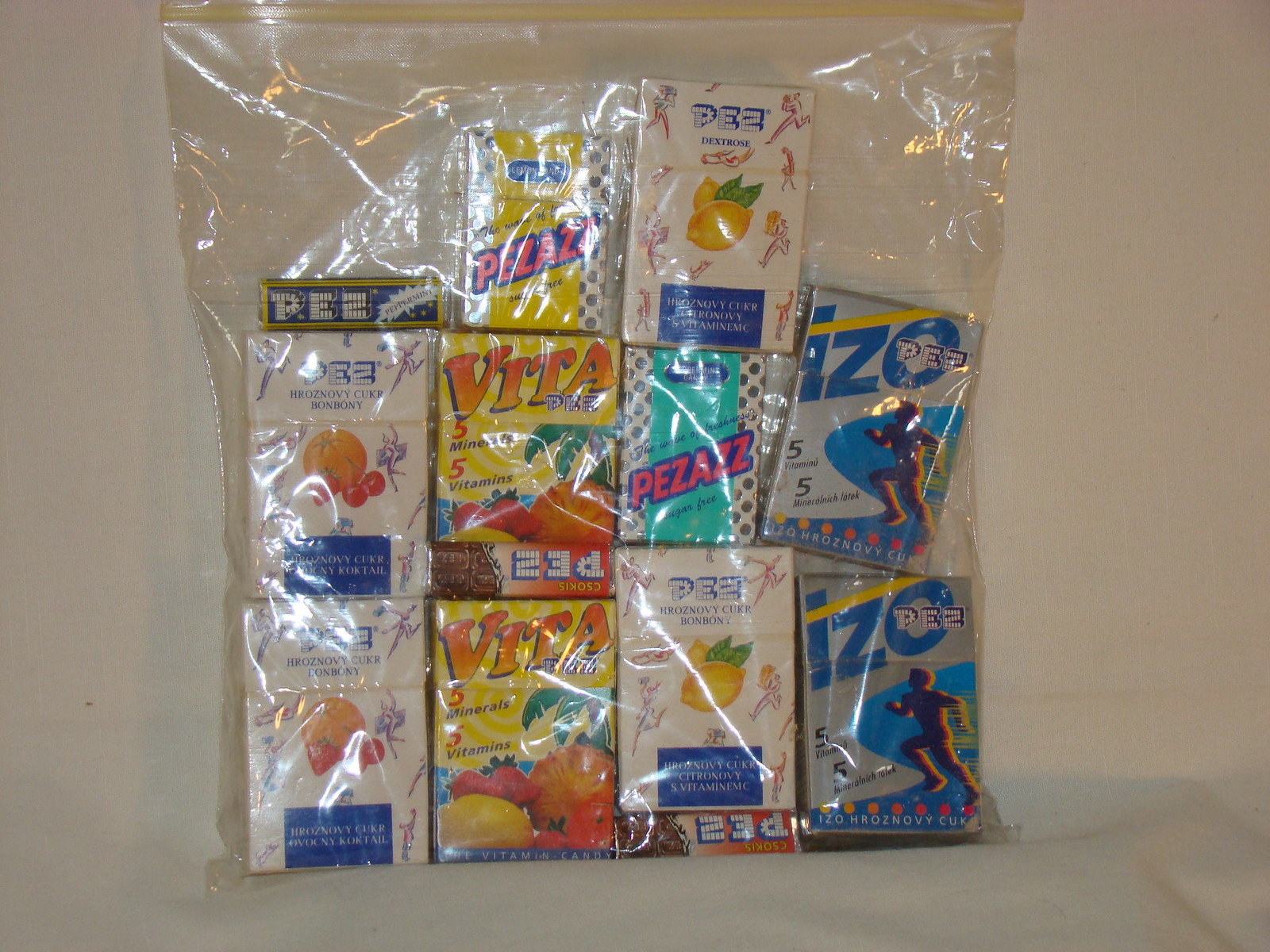This photograph features a large, completely see-through Ziploc bag, standing upright against a white wall and resting on a white linen cloth. Inside the bag are neatly organized rectangular packages of Pez candies. Dominating the view within the bag are multiple rows and columns of colorful Pez packaging. Prominently displayed are several yellow packages branded as "Vita" with orange gradient block letters and small fruits depicted on the front, indicating they contain vitamins. Accompanying them are a few Pez packages with blue and white lettering spelling out "P-E-Z." Additionally, there is a distinct gray package labeled "IZO" with blue block letters and a silhouette of a running person with yellow speed lines trailing behind him. Altogether, the packaging creates a visually organized array of bright and colorful candy boxes within the transparent bag.